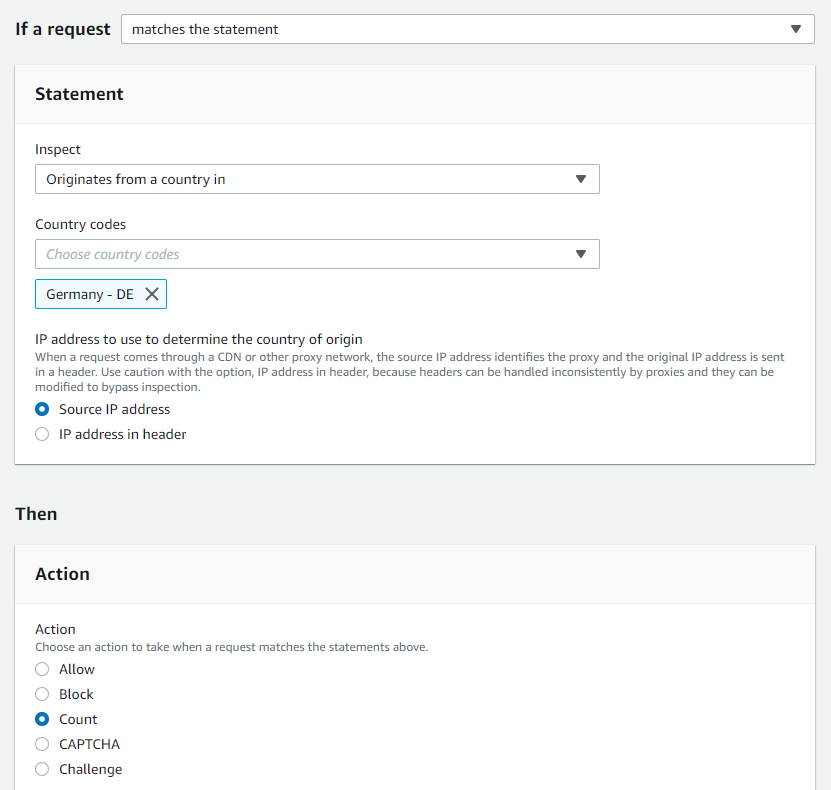The image depicts a gray interface box containing several interactive elements designed for refining request criteria and subsequent actions. At the top, a drop-down menu is visible, labeled "If a request." The selected option in this menu reads "matches the statement," displayed in black lettering. 

Below, a larger box labeled "Statement" includes another interactive drop-down, labeled "originates from country," from which "Germany - DE" is selected and highlighted in blue. A note underneath explains, "IP address to use to determine the country of origin," and provides further clarification that requests coming through a CDN or proxy network will have source IP addresses identifying the proxy while the original IP address is included in a header. A caution advises careful use of the "IP address in header" option due to potential inconsistencies and manipulation risks by proxies.

Two options are provided to define the IP address source: "Source IP address" and "IP address in header," with "Source IP address" selected, indicated by a blue radio button.

Further below, another box titled "Then" contains a smaller label, "Action," prompting the user to choose an action to take when a request matches the aforementioned statements. The available actions are "allow," "block," "count," "capture," and "challenge," with "count" being the currently selected option.